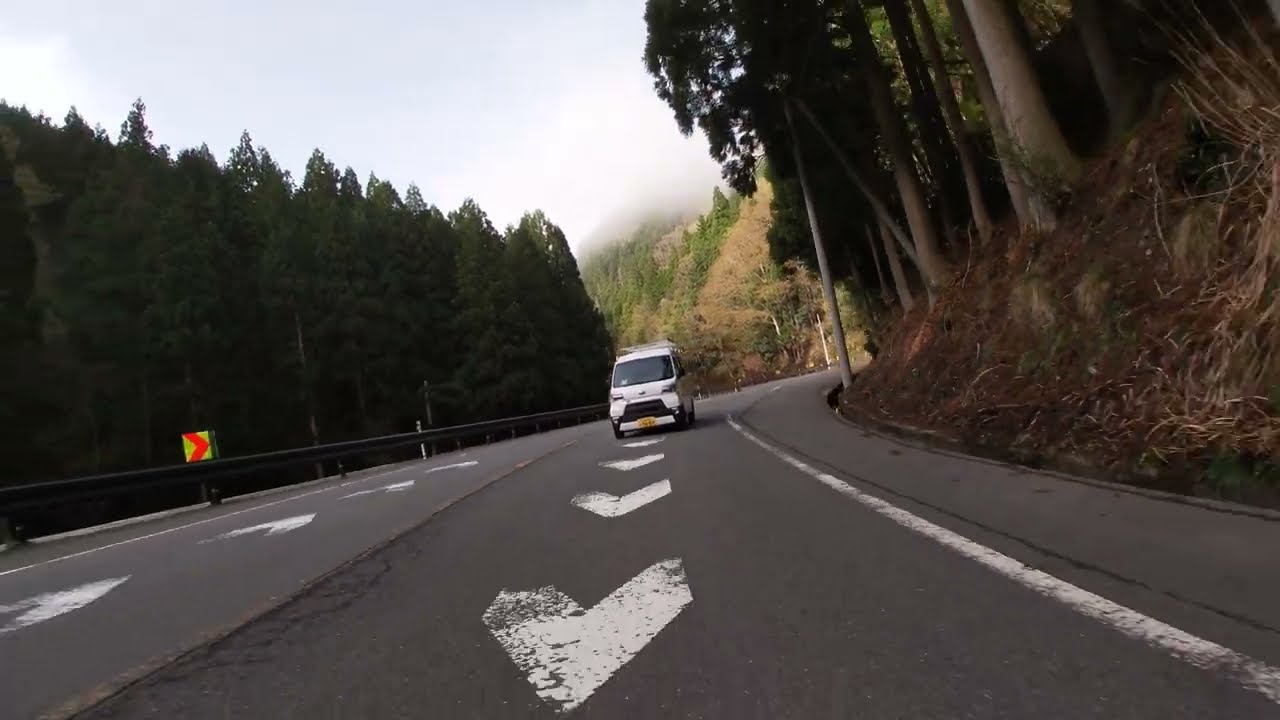This image is a highly detailed photograph of a curving mountain road in a landscape orientation. In the center of the picture, a white van with a black front and a small yellow license plate drives toward the viewer along a dark gray, paved two-lane road. The lane closest to the viewer features large white directional arrows pointing towards the viewer, repeating from the van down to the bottom of the image. The adjacent lane to the left of the van has white directional arrows pointing away into the distance and is bordered by a guardrail with a yellow sign displaying an orange arrow pointing to the right.

On the left side of the road, a densely packed copse of tall coniferous trees casts heavy shadows, creating a dark, secluded atmosphere. In contrast, the right side of the road features a steep dirt hill adorned with various large trees and green-leaved plants. In the background, more forested mountain hillsides and mist-shrouded peaks stretch into the distance, adding depth to the scene.

Above, the sky is a light blue, subtly hinting at daytime, though scattered clouds also seem present, according to some descriptions. The overall visual is a blend of photographic realism, capturing a dynamic and serene mountain environment with a clear focus on the van approaching the viewer along the winding road.